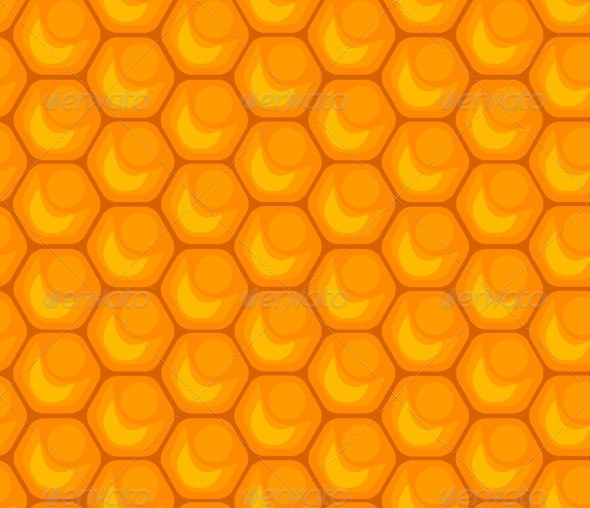This square image features a meticulously arranged pattern resembling a honeycomb, made up of hexagonal shapes. The outlines of each hexagon are a dark brownish-orange, while the interiors showcase a lighter orange hue. Inside each hexagon, there are yellow crescent moon shapes and lighter orange circles, creating a visually engaging, repetitive design akin to Pac-Man figures poised to consume dots. The hexagons are separated by thin lines, highlighted with darker brown tones, adding a spatial distinction between the shapes. A subtle criss-cross pattern of dashed white lines overlays the entire image, contributing to its intricate texture. Additionally, there is a watermark that reads "Envato" spread across the image, ensuring its authenticity. No people or other text are present, allowing the geometric symmetry and the detailed play of colors to dominate the scene.